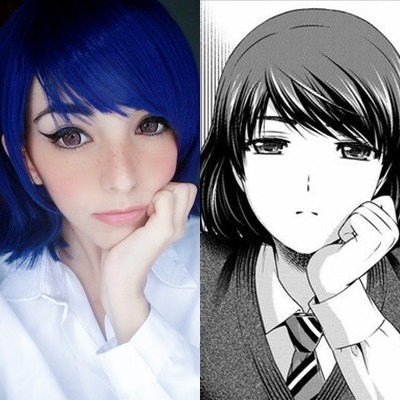The image is a small, square photo split into two sides. The left side features a highly idealized, possibly photoshopped portrait of a young woman, viewed from her upper torso to the top of her head. She has striking blue hair with bangs that nearly touch her brown eyes, and clear, flawless skin, suggesting she might be of Asian descent. Her chin rests on her left hand, and she's wearing a collared, button-down white shirt, although only part of her chest and head are visible. 

The right side of the image displays a black and white cartoon caricature of the same woman. This animated version shares her distinctive blue hair and similar facial features but with a few differences. The cartoon's head is tilted more upright, and she wears a school uniform consisting of a collared shirt, a tie, and a gray sweater vest, differing from the white shirt on the left. Her eyes in the cartoon appear gray with black makeup, and the background is gray with black lines, contrasting the black background on the left. The animated figure's left hand also rests on her chin, mirroring her pose in the real-life photo.